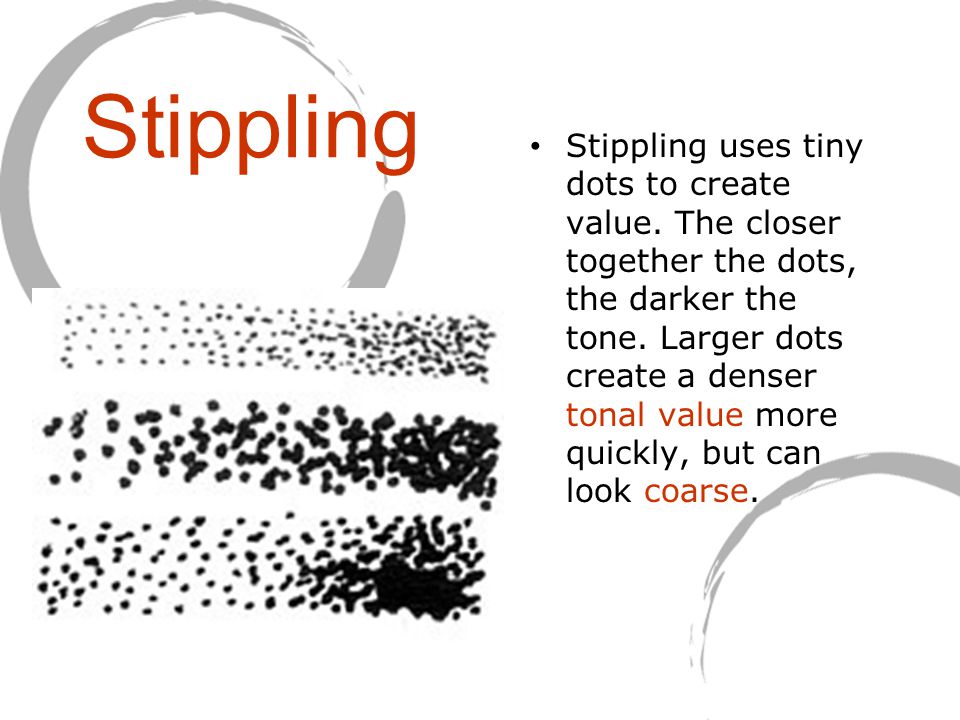The image features a white background with several elements arranged to illustrate the concept of stippling. In the top left corner, a red inscription reads "stippling," framed by a half-circle grey outline. Beneath this, there are three rows of black dots varying in size; the top row starts with finer dots and transitions to larger ones, followed by two more rows of generally thicker dots. On the right side of the image, a black paragraph provides explanatory text: "Stippling uses tiny dots to create value. The closer together the dots, the darker the tone. Larger dots create a dense tonal value more quickly but can look coarse." Notably, the phrases "tonal value" and "coarse" are highlighted in red. At the bottom right, there's a quarter-circle grey outline, subtly balancing the design. The overall arrangement resembles an educational slide, possibly from a PowerPoint presentation, showcasing the visual and instructional use of stippling techniques.